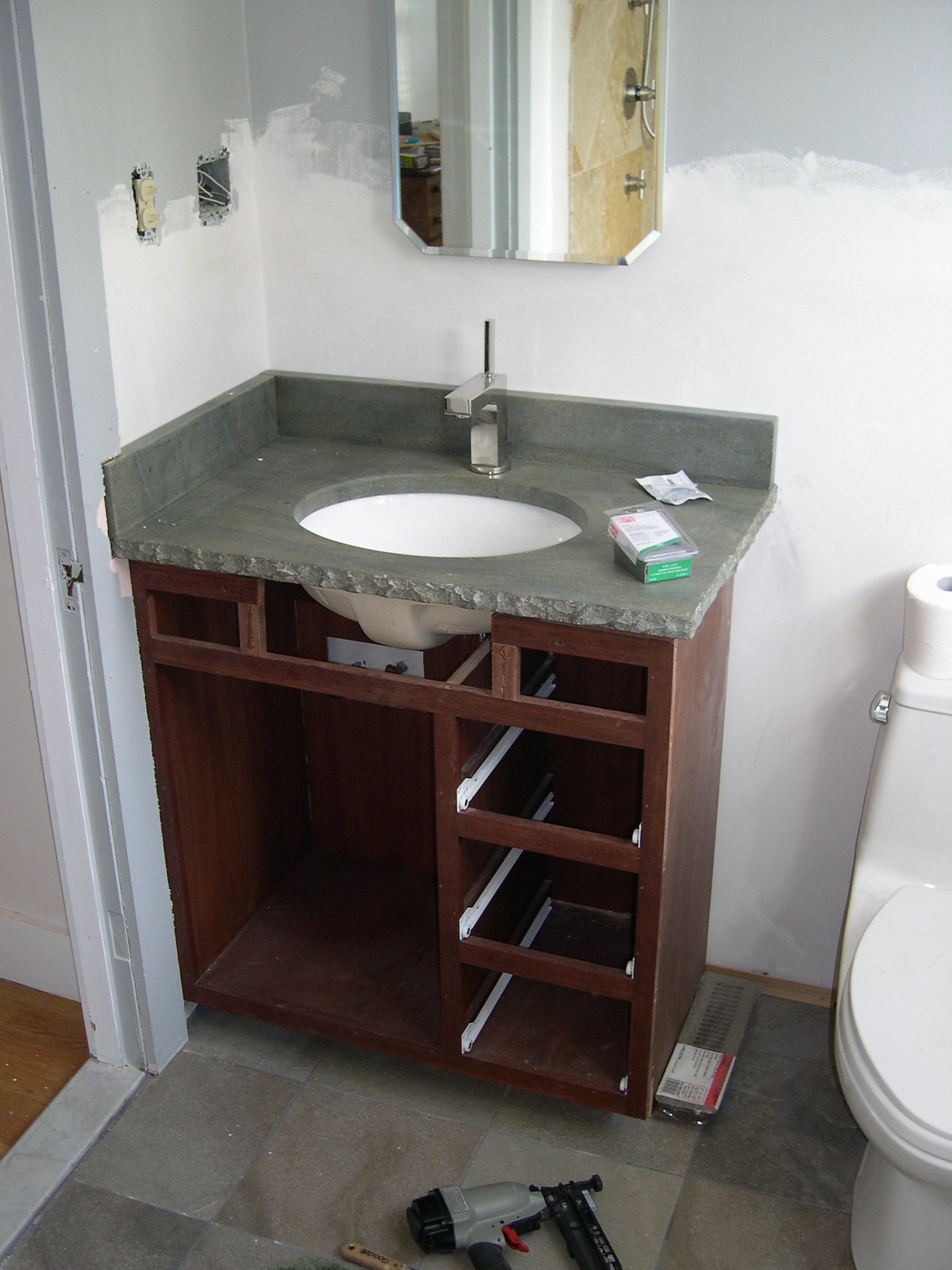The photograph depicts a bathroom undergoing remodeling. Central to the image is a partially assembled vanity featuring a small cabinet designed to accommodate five drawers—a trio of larger drawers are stacked vertically on the right, with two smaller compartments flanking the sink that may eventually house additional drawers. To the left, there is a large opening intended for a cabinet door.

The countertop is made of green marble, characterized by its unfinished, rough edges along the front and side. The wall behind the vanity has been prepped with a coat of white primer on the upper section, while the lower portion remains a neutral gray. Above the vanity, a modern, chrome faucet is installed over an inset, rimless sink set flush into the approximately one-inch-thick marble surface, which also forms the backsplash.

A slender mirror is mounted directly on the wall above the vanity, contributing to the sleek, contemporary design of the space.